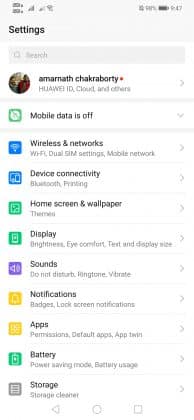This is an image of a smartphone settings screen, albeit quite blurry. At the top, the screen displays the title "Settings." Below this, the name "Amarnath Chakraborty" is visible, followed by "Huawei ID, Clock, and others." There is an indication that the "Mobile Data" is turned off.

Moving further down, a section header titled "Wireless & Networks" is visible, listing options such as "Wi-Fi," "Dual SIM settings," and "Mobile network."

Following this is the "Device Connectivity" section, featuring options like "Bluetooth" and other indistinguishable words due to the blur. The next section appears to be titled "Home Screen & Wallpaper," though some words are not clearly legible.

The "Display" section follows, showing settings like "Brightness," "Eye Comfort," and another unreadable option. Below this, the "Sounds" section includes "Do Not Disturb," "Ringtone," and "Vibrate."

There's a section for "Notifications," which covers settings like "Badges" and "Lock Screen Notifications." Finally, the "Apps" section is listed at the bottom of the screen.